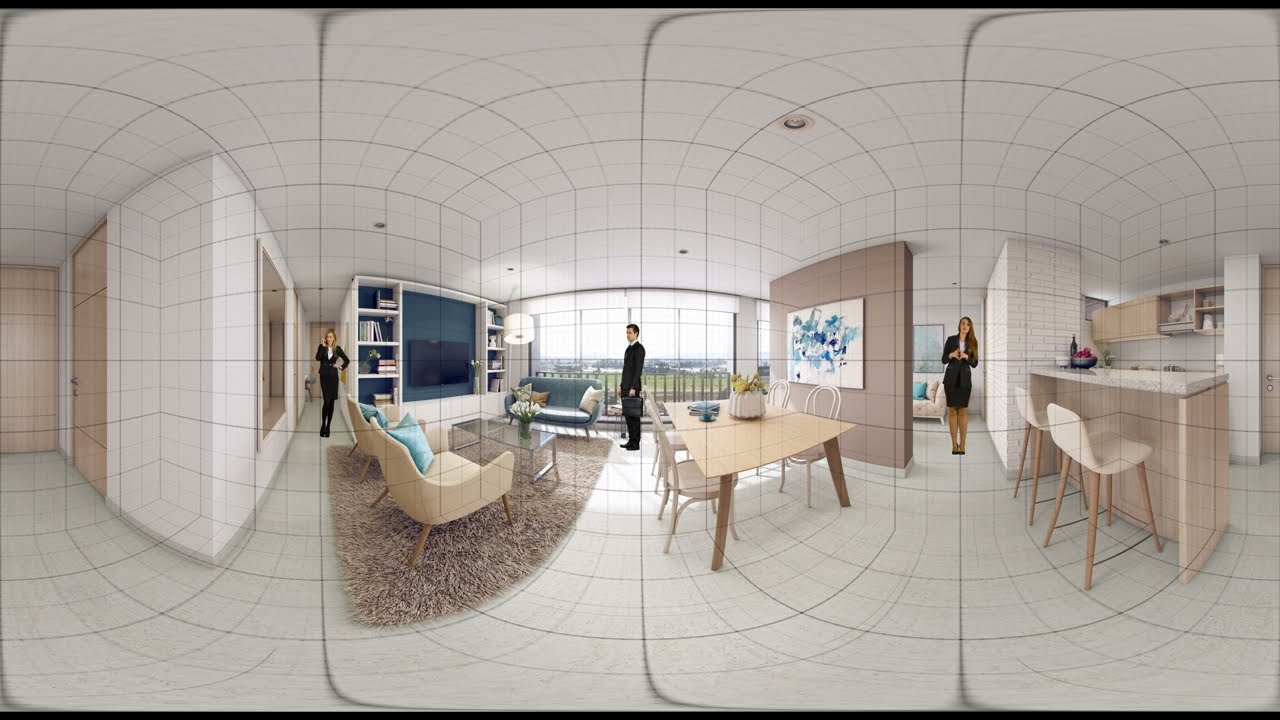The image depicts a luxurious, open floor plan apartment characterized by a sophisticated, post-modern design. It exudes high-end elegance with its soft white and tan color palette, featuring white walls, ceilings, and floors complemented by tan doors, furniture, rugs, and a dining table with chairs. In the living area, a greenish couch and white chairs with blue and white pillows add a touch of color. A large black TV is mounted on the left wall, surrounded by white bookshelves.

Prominent within the space are three individuals dressed in professional black attire: a woman in a black suit stands to the left near the entrance hall; a man in a black suit with a white undershirt stands at the center; and another woman in a black dress is situated between the living room and kitchen area. The kitchen features a white countertop, white chairs, and stainless-steel appliances, and includes a tan bar section with matching stools.

Additional details include large windows that reveal a cloudy day outside, a brown wooden table accompanied by white chairs, and an art piece with shades of blue and black on a gray wall in the center of the room. The entire scene is overlaid with curving black lines, giving it a graph-like appearance that sections the room in a visually unique manner.